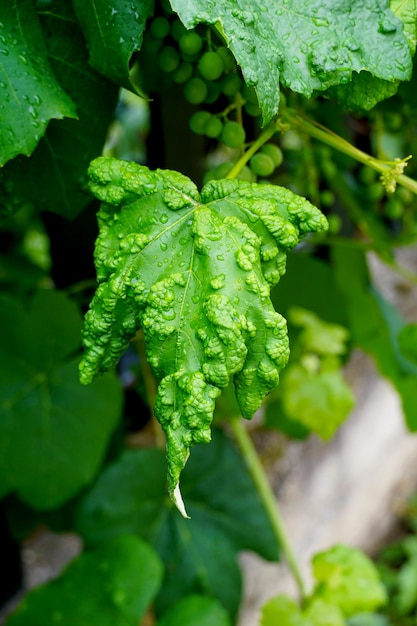This nature photograph features an extreme close-up of a bright green leaf, likely from a grapevine, covered in water droplets, suggesting recent rain or dew. The leaf is distinctive due to its textured surface, adorned with raised, green, wart-like growths scattered across it. Some interpretations suggest these might be natural formations, some type of fungus, or even larvae. The leaf's intricate details, including its rough surface and bright, pea-shoot green color, dominate the image. In the background, slightly out of focus, more leaves and green grape clusters can be seen. There are also green stems and a vague, whitish structure, potentially a tree trunk or a container, adding further complexity to the scene. The overall composition highlights the wet, fresh ambiance of early morning or post-rainfall.